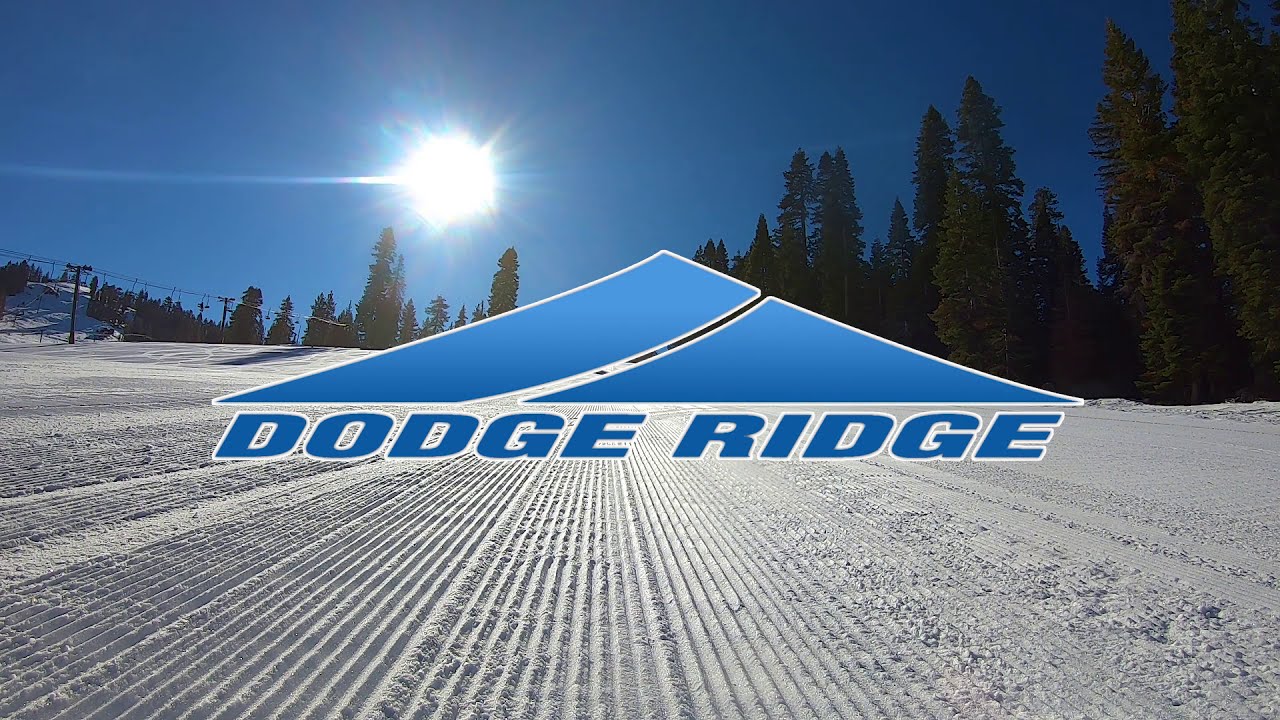This is a highly detailed outdoor photograph reminiscent of an advertisement. It features a sunlit ski slope blanketed in snow that has been meticulously graded, creating a corrugated pattern. Surrounding the snow-covered field are towering evergreen pines, forming a natural boundary. To the left, a ski lift and telephone pole with wires are faintly visible in the background. The scene is illuminated by a brilliant sun set in a bright blue sky. Prominently displayed in the center is a blue logo depicting a mountain-like triangle, with the words "Dodge Ridge" in blue, outlined in white situated below the symbol.